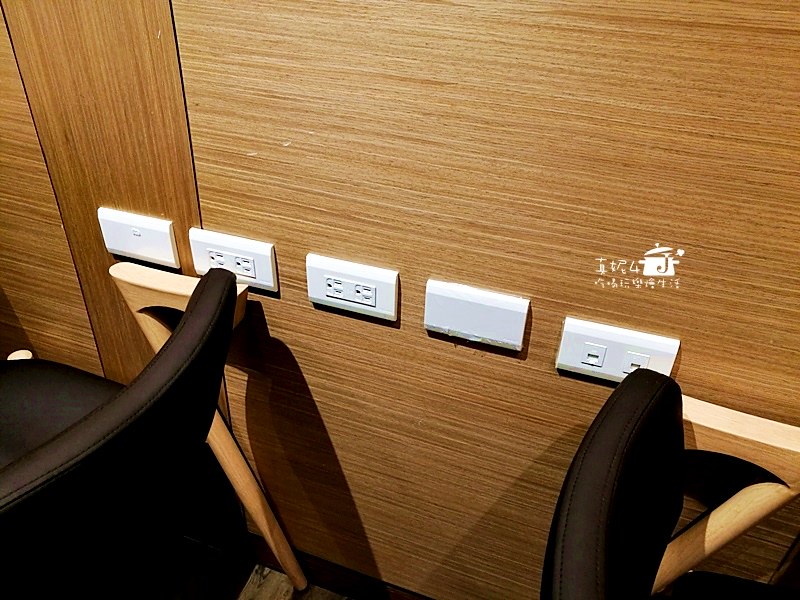The image depicts a wall with wooden paneling, characterized by a diagonal grain pattern. Central to the composition are five wall outlets arranged diagonally. The first outlet is a switch, the second and third are twin electrical sockets, the fourth appears to be an old-fashioned phone jack, and the fifth is an outlet with two switches. Above the fifth outlet, there are Japanese symbols or text. The wall has a warm brown hue, and along the bottom and side of the image are chairs featuring dark brown fabric and black leather backings, with wooden armrests and legs. The setting suggests it could be a restaurant, given the arrangement and nature of the furnishings.